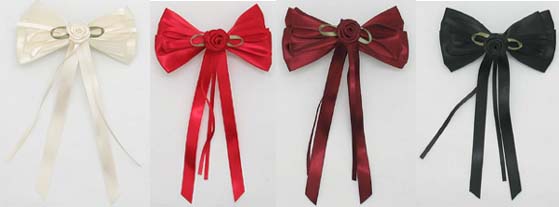The photograph displays a horizontal rectangular image divided into four equal sections, each featuring a differently colored bow set against a stark white background. From left to right, the bows are white, bright red, deep maroon, and black. Each bow follows the same intricate design: a bow tie shape at the top with a small rosette in the center, crafted from the same fabric, surrounded by a gold trim. Long ribbons hang down from each bow, comprising two wide and two thin strips, all matching the color of the respective bow. This consistent styling across the four bows, coupled with the plain background, highlights the subtle differences in color and the delicate details of each ribbon and rosette.